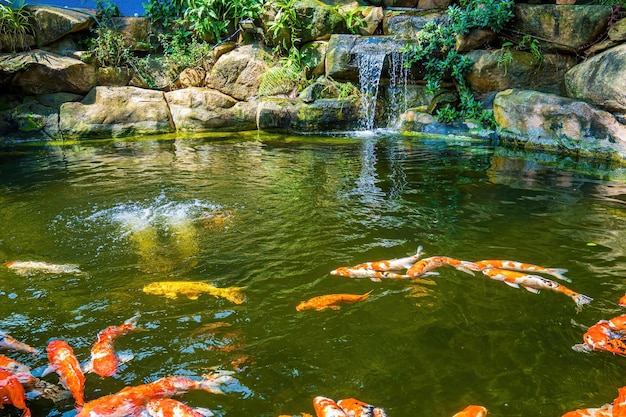This image features an outdoor scene of a serene lagoon or pond with greenish water, teeming with vibrant koi fish in shades of orange, yellow, and white. Sporadically swimming around, these fish create occasional splashes, one of which is discernible toward the left middle of the pond. Dominating the background are large, gray rock formations interspersed with lush, dark green vegetation that drapes down their sides. Among these rocks, on the upper right-hand side, a small, gentle waterfall cascades over its own rocky perch, adding to the tranquil ambiance as it splashes into the pond below. The rocks extend from the upper left across the image, tilting slightly downward to the right, with some rocks on the far right featuring distinctive white and black markings. The koi fish are scattered throughout the pond, with notable clusters of orange and white fish visible in both the bottom left and right corners, gliding gracefully beneath the water's surface and occasionally breaking through it.